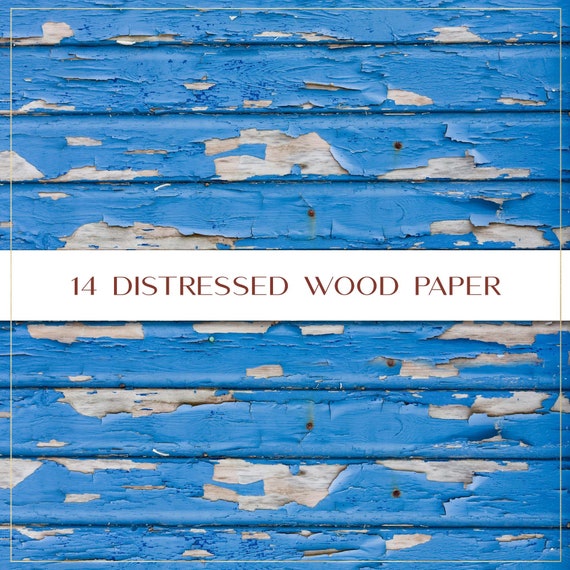The image depicts a weathered, beachy-blue background that mimics the appearance of distressed slatted wood, with visible signs of peeling paint revealing patches of gray and brown underneath. The backdrop consists of multiple horizontal sections of wood, highlighting the rustic texture. A thin white rectangular border frames the entire image, adding to its structured appearance. At the center of the image, spanning horizontally from left to right, is a prominent white rectangular banner. The banner features the text "14 distressed wood paper" in brown font, signifying either a product advertisement or scrapbook paper. The overall look gives a sense of aged, weather-beaten wood, ideal for creative projects like scrapbooking, especially with a beach or rustic theme.